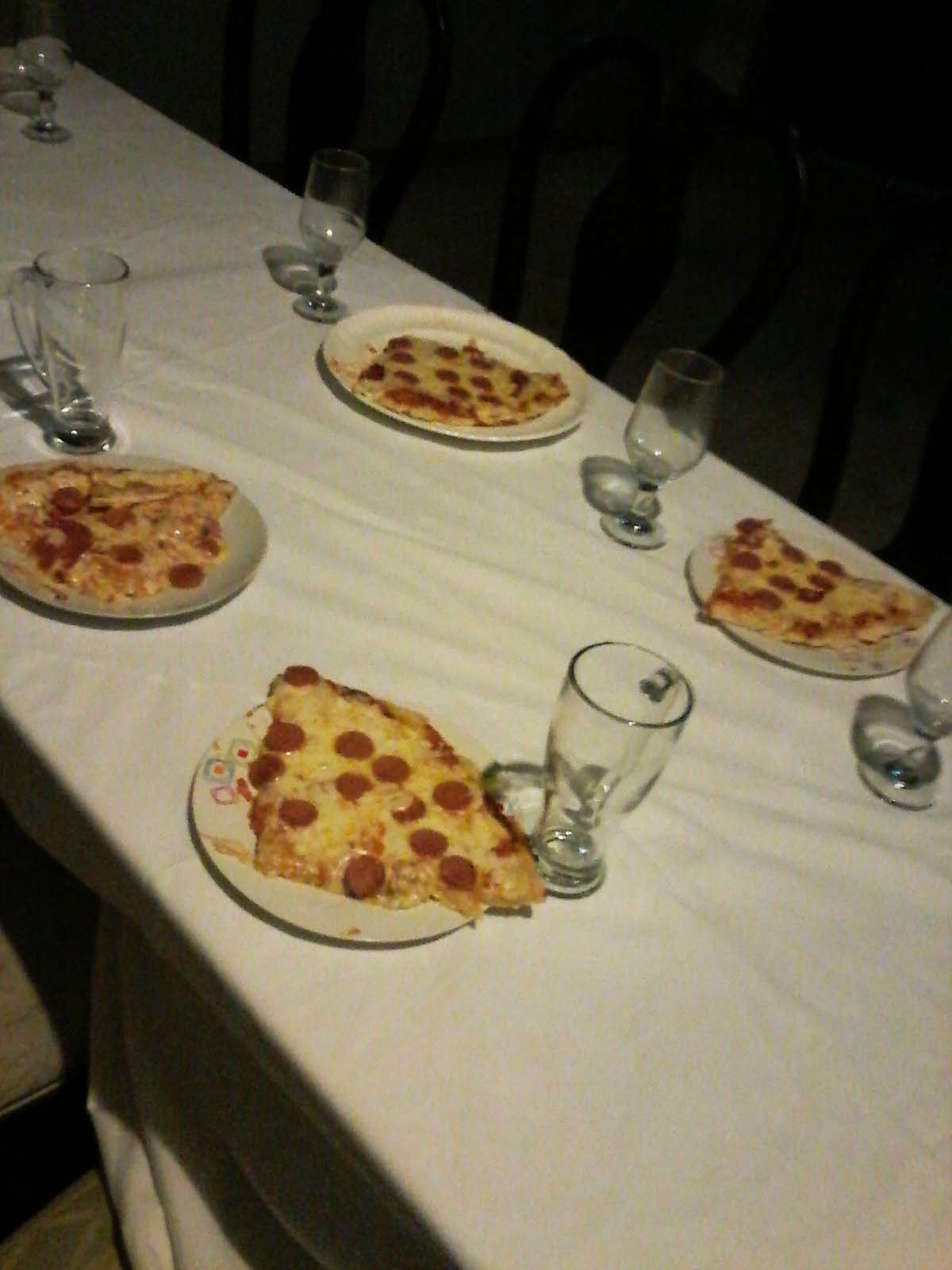The image is an angled, overhead view of a long table draped in a white tablecloth, which cascades to the floor, where it appears bunched up in the bottom left corner, partially revealing a gray chair cushion. The tablecloth, slightly wrinkled, supports four white ceramic plates adorned with minimal geometric designs, partially obscured by the generous slices of pepperoni pizza atop them. Each plate holds two conjoined pepperoni slices, their melted cheese oozing over the edges, and the plates themselves appearing too small, causing the pizza to hang off the sides on some.

Adjacent to each plate sits a tall, clear glass—two resembling beer steins with handles on the left side and two more like elegant goblets on the right—all devoid of any liquids. The photograph captures a stark contrast between the brightly lit table and the dark, nearly black background, which features faint, indistinguishable lines suggesting a patterned backdrop and an obscured view of chairs beneath the table. The overall image exudes a cozy yet slightly disarrayed ambiance, emphasizing the delectable appearance of the pepperoni pizza against the otherwise dark and undefined setting.